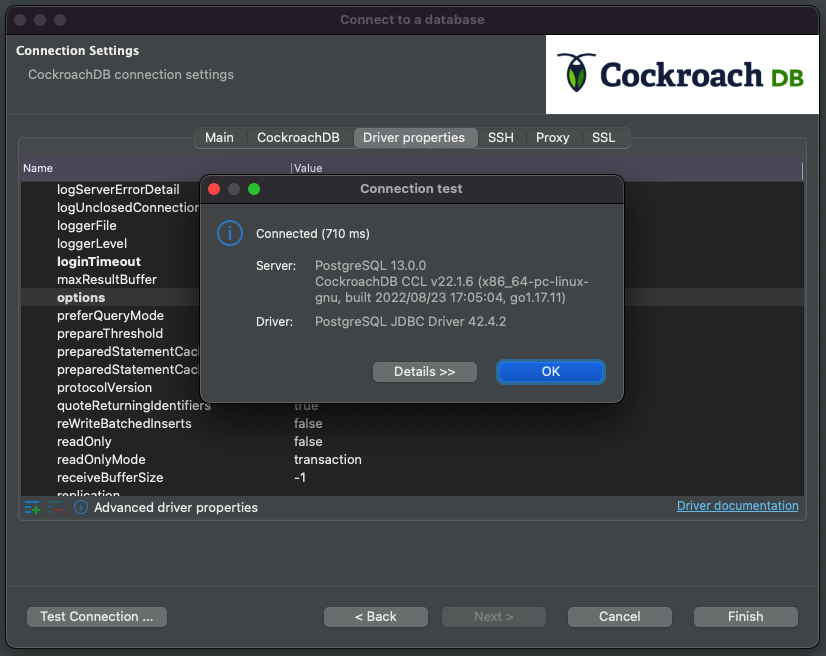The image depicts a screenshot of a database connection interface. The background is predominantly grey, with a black bar across the top that centrally displays the text "Connect to a Database." Below this is a grey section, which on the left side features the heading "Connection Settings" followed by "CockroachDB" written prominently in large letters.

On the right side of this section is a white box with "Cockroach" written in blue letters in the center, accompanied by "DB" in green letters. An image of a cockroach with a blue outline and blue-green body is positioned in front of these words.

Beneath this, in the center, there is a list of options in white text: "Main," "CockroachDB," "Driver Properties," "SSH Proxy," and "SSL." To the left of this, there is another list labeled with "Name" and "Logs Server Error Detail," under which further information is itemized.

Overlaying this interface is another box with a black bar at the top marked "Connection Test." On the left side of this box are three circles: a red one, a grey one, and a green one. The central area of the box is grey and contains a blue circle with an eye icon, beside the text "Connected 7110ms." This section also includes detailed information about the server and driver. There are two buttons at the bottom of this overlay: a grey "Details" button and a blue "OK" button, with additional information extending below.